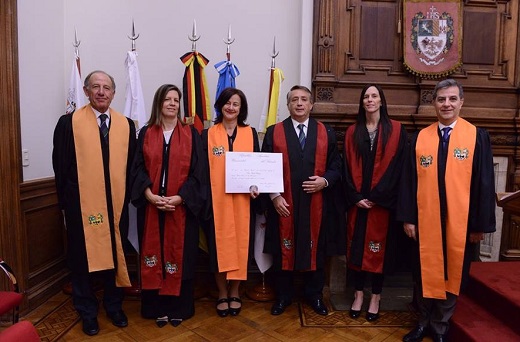In this detailed image, six adults, three women and three men, are captured in what appears to be a solemn yet joyous graduation ceremony held in an ornate, wood-paneled room suggestive of a prestigious UK university. Behind them, a grand wooden mantel adorned with a prominent heraldic crest sets the distinguished tone of the setting. The group stands before four folded flags positioned to their left.

The individuals are all dressed in formal attire, enhanced by ceremonial robes and sashes that correspond to their gender—orange sashes for the men and red sashes for the women. The man on the far left, a distinguished older gentleman, sports a black suit with a white shirt and black tie, accented by an orange shawl draped down to his shins. Beside him, a woman with shoulder-length hair wears a black robe and red shawl. In the center, a dark-haired woman, joyfully holding up a certificate, is dressed in a similar black robe but with an orange shawl. To her right, another gentleman, approximately 45 years old, stands with hands at waist height, dressed in a black suit with a blue tie and red shawl. The penultimate figure, a slender woman with long black hair, matches her female peers in a black robe and red shawl. Completing the lineup, another man, possibly in his early 50s, is seen slightly stepping forward with short hair, a white shirt, blue tie, and an orange shawl over his black robe.

The celebratory atmosphere is palpable, as all six individuals wear bright, proud smiles, clearly marking a significant achievement or occasion.